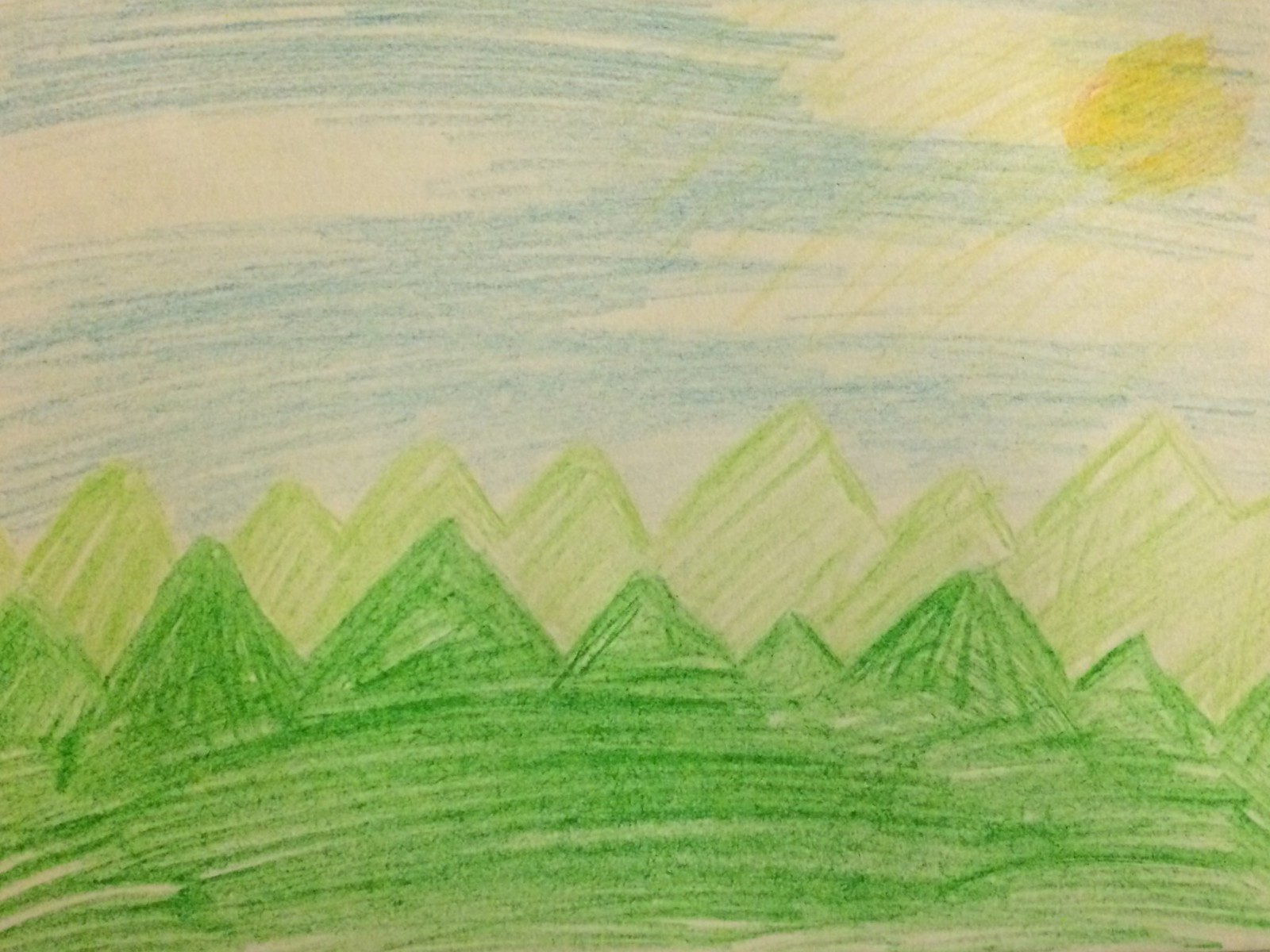This vibrant child's crayon drawing depicts a picturesque mountain range scene. At the bottom, a lush, green foreground made up of horizontal streaks of varying shades of green suggests rolling grass. Behind the grassy field rise seven pointed, triangular mountains of different sizes, creating a striking silhouette against the sky. The two mountains on the far left are identical in height and resemble equilateral triangles. Further right, the peaks decrease and increase in height, forming a dynamic and varied landscape with the shortest peak being the fifth from the left.

The mountain range is portrayed in a pale green hue, with the crayon strokes applied diagonally at a 45-degree angle leaning to the right, giving the mountains a textured appearance. Despite the visible crayon strokes, the mountains are not fully filled in, adding a whimsical, unfinished charm to the artwork.

In the upper right corner, a bright yellow sun beams down, interspersed with curious blue streaks that create an intriguing contrast. The sky above the mountains is a collection of horizontal blue streaks, with deliberate gaps left white, evoking a partly cloudy sky.

Together, these elements create a lively and imaginative representation of nature through the eyes of a child, rich with color and energy.